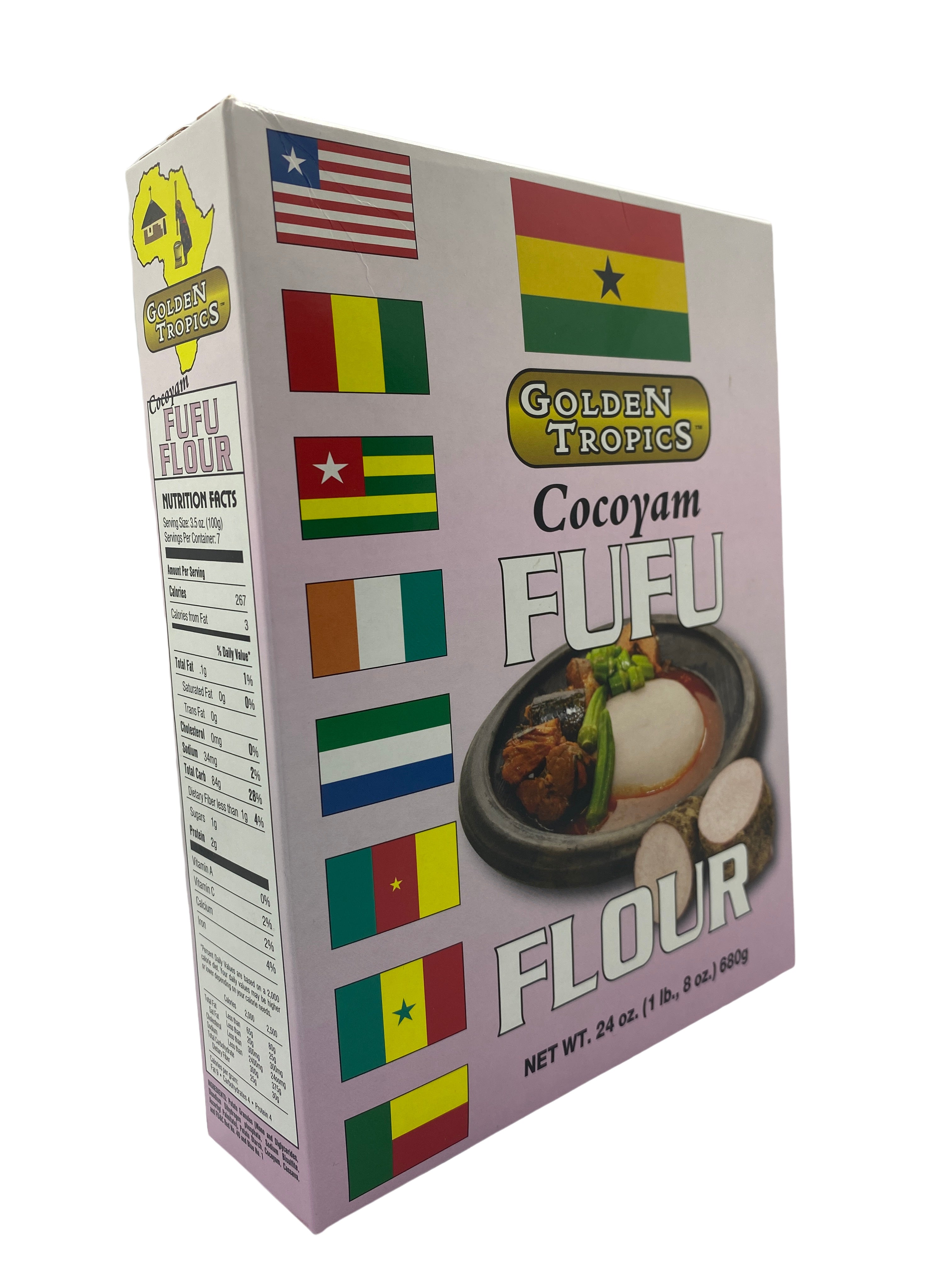The image presents a packaging photograph of a product called Fufu Flour by Golden Tropics. The cardboard box, angled to show its front and left side, is primarily lavender with a hint of pink. "Golden Tropics" is prominently displayed within a rounded-edged, golden rectangle both on the front and left side, accompanied by the brand's logo: a map of Africa with a building and a statue within it. Nine flags of various African nations adorn the packaging—one large one at the top center above the logo, and eight smaller ones descending along the left edge of the front panel.

Below the brand name on the front, "Coco Yam" is written in black print, followed by "Fufu Flour" in bold white letters outlined in black and blue, separated by an image of a traditional African dish resembling mashed potatoes and stew. The net weight, although partially obscured, suggests the package holds over a pound of flour, possibly around 24 ounces. The nutritional information is listed in a white panel along the left side, formatted similarly to U.S. standards. The primary focus of the elaborate design and multiple flags underscores the product’s connection to African heritage and cuisine.